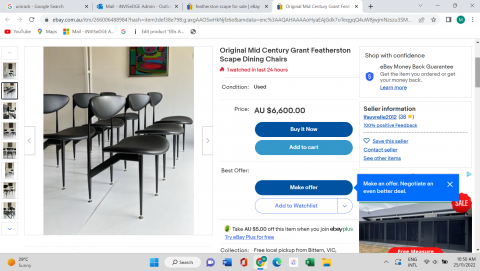This image appears to be a screenshot taken from a website, possibly an e-commerce platform. At the top, there is a thin gray navigation bar with four tabs—the first three are gray while the fourth one is white. The first tab displays a company icon to the left, followed by text that is too blurry to decipher. Directly below this bar, there is a search bar with unreadable text and a green circle on the right side featuring a white letter "M."

Beneath the search bar is another navigation strip that includes icons for YouTube, Google Maps, and email, along with the Google Home icon. The associated text for these icons is also indiscernible. On the left side of the page, there is a column displaying nine small images of black chairs arranged in a room.

The right side of the page features a larger image depicting a room with a tan wall and a white floor. A colorful, abstract painting hangs on the back wall. The room contains six chairs, three positioned from right to left in the foreground and another three arranged behind them to the left. To the right of this main image, there is black text stating "Original Mid-Century Brand Featherstone," followed by "Escape Dining Chairs" in smaller text beneath it. In red text, it is noted that one of these chairs has been ordered within the last 24 hours. 

Below this text, there is a listed price and three buttons: a dark blue "Buy It Now" button, a light blue "Add to Cart" button, and another blue button labeled "Make an Offer." Additionally, there is a white button labeled "Add to Watch List."

Running down the right side of the page, there is text that reads "Shop with Confidence," followed by information concerning eBay's guarantee and seller details. There are clickable tabs for contacting the seller and viewing other items. In the bottom left corner of the page, there is an image of the exterior of a white building enclosed by a large black fence.